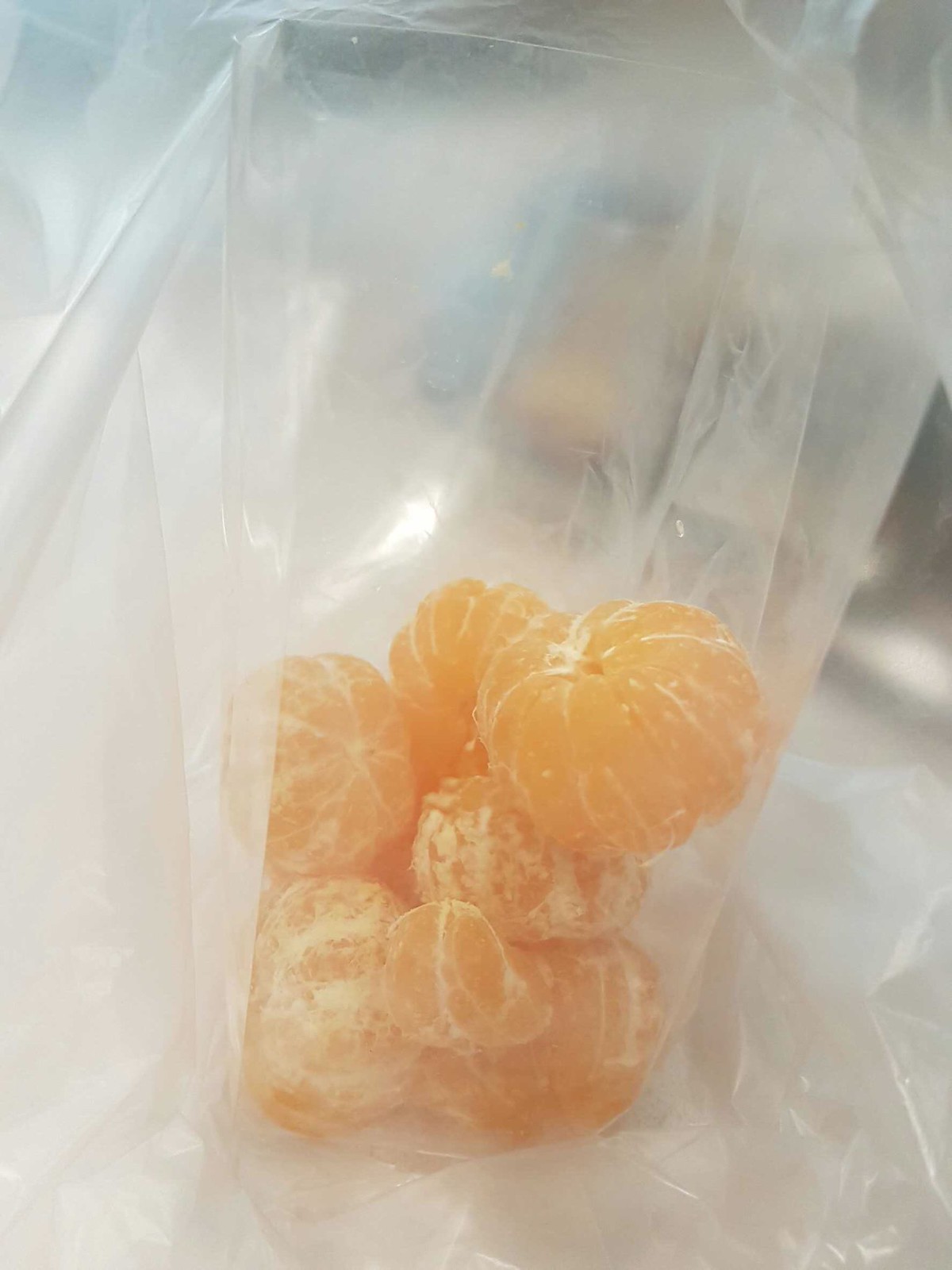This image is a detailed photograph of several peeled segments of citrus fruit, likely mandarin oranges, tangerines, or similar small varieties like cuties, placed inside a translucent plastic or cellophane bag. The vibrant and light orange-colored fruit segments appear fresh, juicy, and plump, indicating they were recently peeled. The segments are clustered together at the bottom of the bag, with some stacked on top of others, and a few still partially covered with the white interior rind. The surface of the plastic bag is smooth and shiny, reflecting light and slightly distorting the view of the fruit inside. This gives the fruit a softly muted, slightly blurred appearance. The bag's interior folds are visible on the left side, with light shining through, suggesting the photo was taken in a brightly lit indoor environment. The focus of the image is clearly on the citrus fruit within the bag, and while the bag and background are subtly indicated, the fruit's fresh and delicious look is the main emphasis of the photograph.